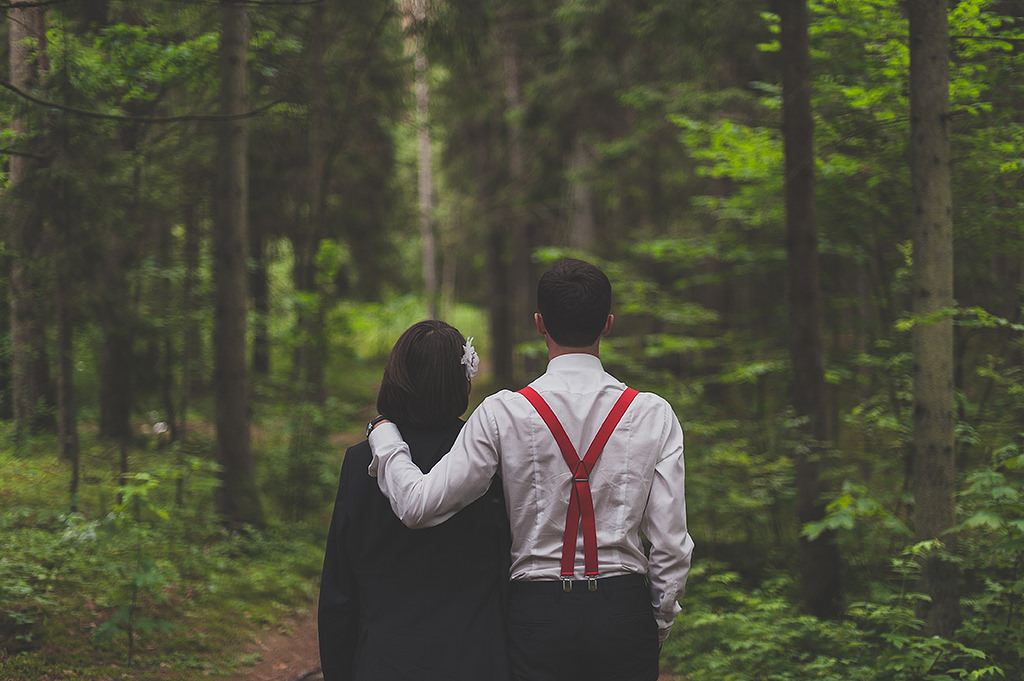In the image, a couple stands in the center foreground of what appears to be a peaceful forest scene. The man, slightly taller with short dark hair, is dressed in a white shirt, red suspenders, and black dress pants. His arm is affectionately draped over the shoulder of the woman standing beside him. The woman, with short brown hair and a white flower tucked behind her right ear, is wearing the man's black or deep blue coat over her own outfit. They are facing away from the camera, gazing into the blurred and somewhat hazy focus of the verdant forest and pathway ahead of them. The contrast between the sharply focused couple and the softly indistinct forest backdrop adds a surreal quality to the photograph, which measures approximately nine inches wide by eight inches tall. This serene moment seems to capture a quiet and intimate walk, with the man offering his coat to the woman, likely to keep her warm.